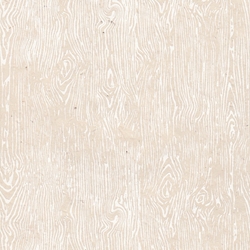The image depicts a small, square, wood grain texture in a very light pink color that appears almost white on the screen, making it challenging to discern. The wood grain pattern runs vertically with intersecting lines and visible knots, resembling the detail one might find on a piece of hardwood flooring. The pattern features delicate, spiral-like streaks with contrasting lighter and darker hues, creating a sense of depth and texture. Despite its subtlety, the texture captures the intricate detail and natural variation found in wood grains.